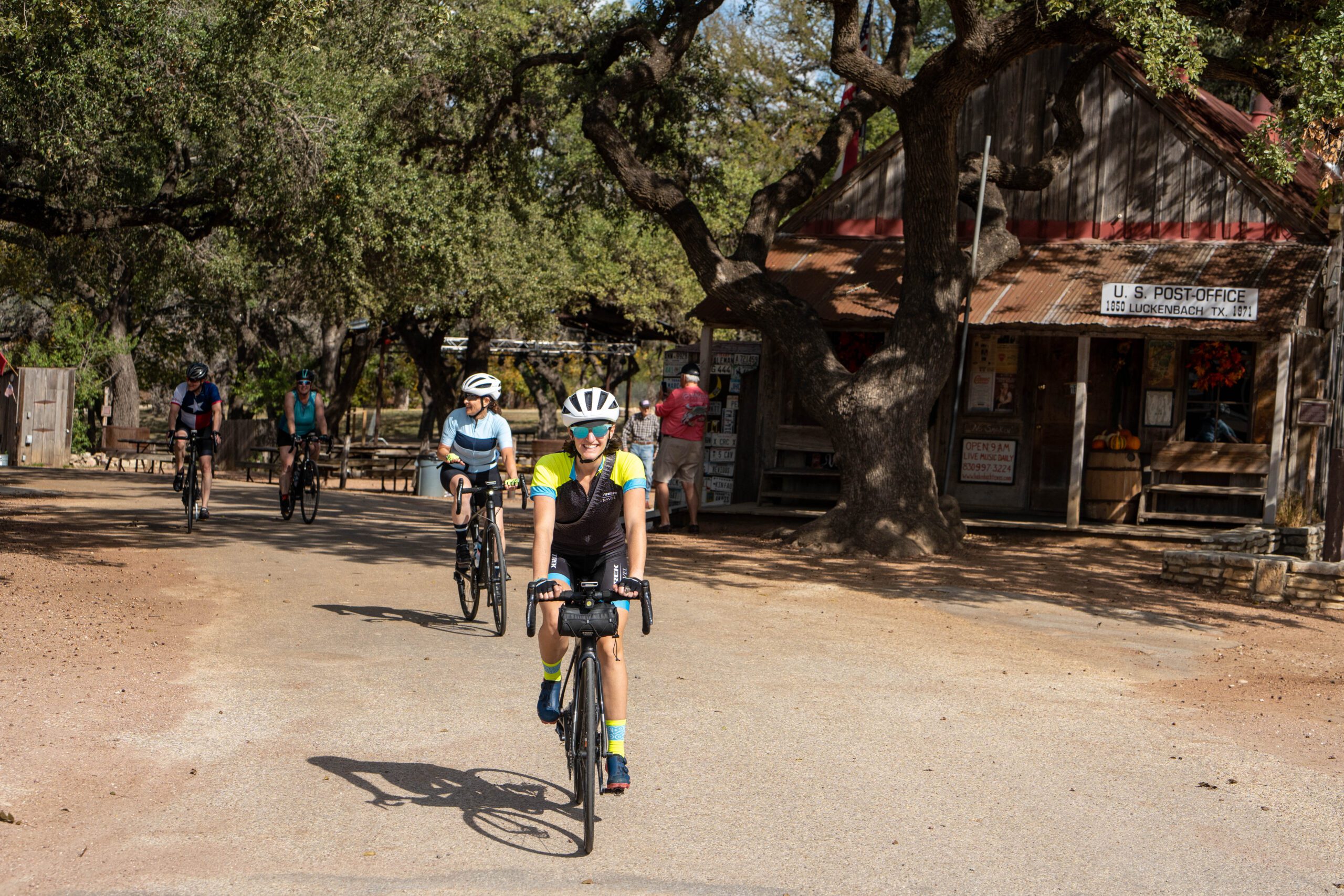The photograph captures an outdoor scene set in the woods, focusing on a group of four bicyclists riding along a dirt road. The central figure is a smiling woman wearing a white bike helmet, sunglasses, a yellow shirt with blue collar and sleeves, and blue shorts. She is riding a black bicycle. Behind her are three more bicyclists, all dressed in sport bike clothing. The background features a rustic building that resembles a log cabin, identified as a U.S. Post Office, likely located in Texas. This post office is partially shaded by trees, with a sign on its roof. To the right of the building and under the dense canopy is a large tree, while the left side of the image is dotted with more trees, pine cones, and hay. Additionally, there are two bystanders near the post office, and further in the backdrop, there is a man walking away. The landscape includes picnic tables and chairs, enhancing the scene’s serene, outdoor ambiance.